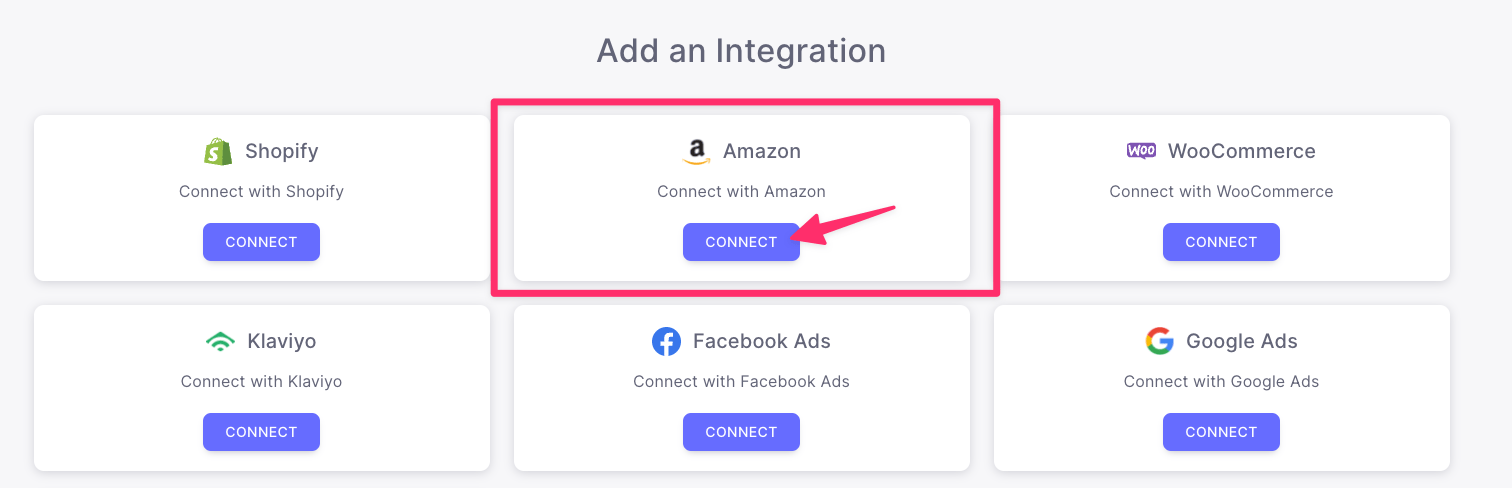This screenshot displays a webpage designed for integrating multiple accounts into a central platform. At the top of the page, the heading "Add an Integration" is prominently displayed in gray text. Below this heading, there are two rows, each containing three integration options.

In the top row, the first option on the left is for Shopify, which includes a label "Connect with Shopify" above a purple "Connect" button. The second option, situated in the center, features Amazon inside a red box. It has a label "Connect with Amazon" and includes a distinctive red arrow pointing toward the purple "Connect" button. The third option on the right is for WooCommerce, similarly labeled "Connect with WooCommerce."

In the bottom row, the first option on the left is for Klaviyo, spelled "K-L-A-V-I-Y-O," with an accompanying label "Connect with Klaviyo" and a purple "Connect" button. The middle option focuses on Facebook Ads and is labeled "Connect with Facebook Ads." The final option, on the right, is for Google Ads and is labeled "Connect with Google Ads."

Overall, this setup allows users to integrate various services and platforms, such as Shopify, Amazon, WooCommerce, Klaviyo, Facebook Ads, and Google Ads, into the main website through the provided "Connect" buttons.